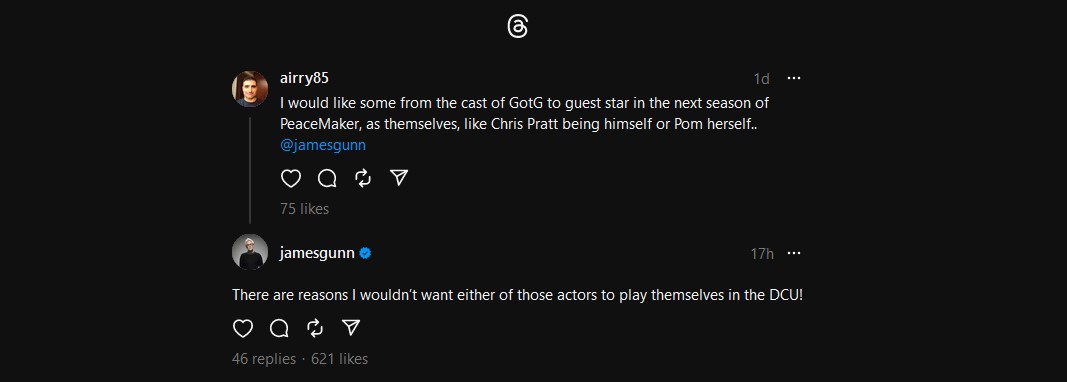**Caption:**

In this image, we see a social media interface reminiscent of Twitter or Instagram Threads. The screen predominantly displays a conversation featuring a younger man identified as Aery85 (username spelled as A-I-R-Y-85). Aery85's profile picture shows a young man with brown hair. One day ago, Aery85 posted a suggestion expressing his desire for cast members from "Guardians of the Galaxy" (GOTG) to appear as guest stars in the next season of "Peacemaker," specifically mentioning Chris Pratt and Pom Klementieff, and tagging director James Gunn. This post garnered 75 likes.

Beneath Aery85's post, there is a response from James Gunn, recognizable by his verified account status and an older gentleman's profile picture. James Gunn replied 17 hours ago, stating that there are reasons why he wouldn't want either of those actors to play themselves in the DC Universe (DCU). This reply has received 621 likes and 46 replies. The interface, resembling Instagram Threads, serves as the platform for this engaging exchange between fans and the director.